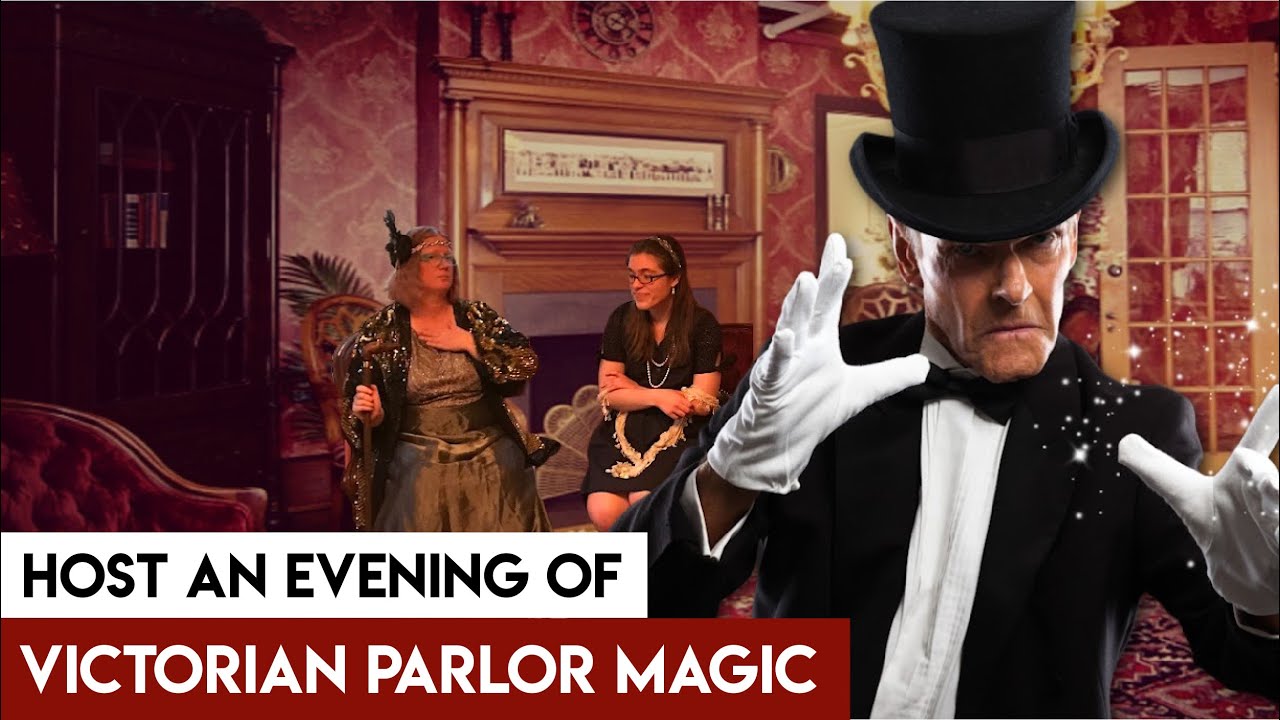The image is a detailed poster titled "Host an Evening of Victorian Parlor Magic." The title "Host an Evening of" is written in black on a white background, while "Victorian Parlor Magic" is depicted in white, all capital letters on a red background. The focal point of the poster is a man in the foreground, dressed in a black top hat, black coat, black bow tie, white shirt, and white gloves. He has just tossed some sparkling glitter into the air and bears a concerned or serious facial expression. Behind him, two women are seated. The woman on the left is dressed in a Roaring 20s style outfit with a side feather in her hair, a half jacket draped over her shoulders, and a baggy dress. The woman on the right sports a more modern look, with a hair ribbon holding back her long brown hair, glasses, a double-strand pearl necklace, and her arms crossed over something in her lap. Her expression is dramatic, adding to the mystique of the scene.